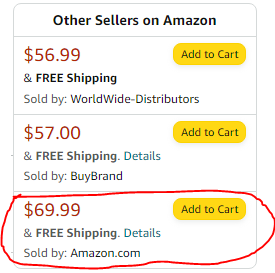The image displays a product listing from a website, featuring various buying options from different sellers. The layout includes a soft grey border with rounded corners and is slightly taller than it is wide. The content is organized into four sections: a thinner top section and three equal-sized sections below.

The top section prominently reads "Other Sellers on Amazon" in bold black font. 

In the first section below, the product is priced at $56.99 and includes free shipping. The seller is "Worldwide Distributors," and there is a yellow "Add to Cart" button.

The second section lists the price as $57.00 with free shipping details. The seller is "By Brand," followed by a yellow "Add to Cart" button.

The final section shows a price of $69.99, also with free shipping details, and is sold by "Amazon.com." This section is notably marked with a red scribbled outline, and includes a yellow "Add to Cart" button.